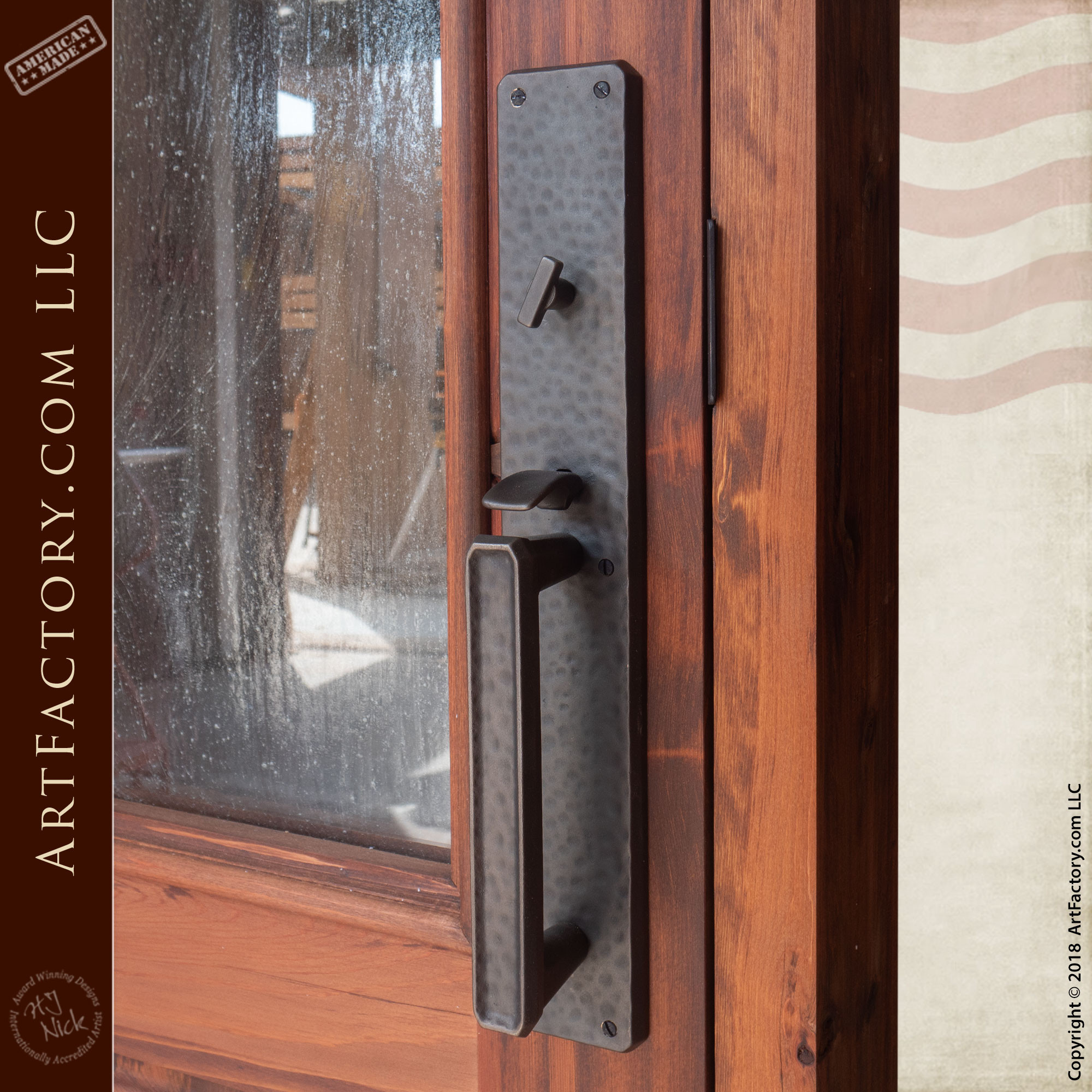This photograph captures an advertisement for ArtFactory.com, showcasing an artisan-quality front door, possibly for a home or office. The door features a medium brownish wood stain and exhibits a sophisticated design with textured glass panes. Highlighting the craftsmanship, there is a heavy, handmade door handle with a distinctive raised alligator print texture. The handle encompasses a metal latch mechanism, further accentuating the door's artisanal appeal. On the left side of the image, the text "ArtFactory.com" is prominently displayed, along with "American Made" and the name "H.J. Nick," indicating the accredited artist associated with the piece. Additionally, the image includes a copyright notice at the bottom right corner, stating "© 2018 ArtFactory.com LLC." The advertisement emphasizes the high-quality, award-winning designs produced by ArtFactory.